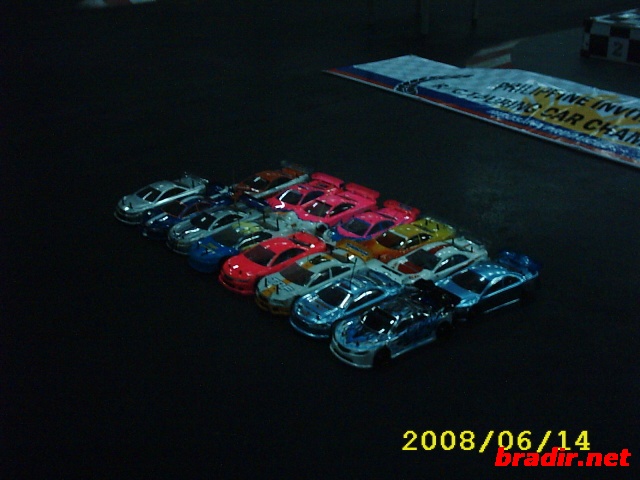A dimly-lit photograph captures an array of toy cars, likely Hot Wheels, meticulously lined up in two rows. The image, which appears to have been taken at night, features cars of various colors, including red, blue, silver, and more vibrant hues. The exact scale of the cars is difficult to discern due to a lack of reference objects. 

In the foreground, the front row consists of a silver car, a dark blue car with a gray stripe, a gray car, a blue car with a yellow hood and door, a red car with a spoiler, another gray car with an orange stripe, a plain blue car, and a final blue car with light blue highlights. The back row showcases an orange car with a white stripe, three pink cars (the third one with blue details), a yellow car with an orange hood, a white car with a red stripe down the center, and a blue car.

The backdrop features a large, white banner with a blue stripe below it and a red stripe beneath that, displaying text that reads "Philippine Invite" and partially visible words "Car Cham," likely referring to 'Champion.' A checkerboard pattern and a number 2 are faintly visible in the distance on the left side but are obscured by the darkness. 

In the bottom right corner, a date, "2008-06-14," is inscribed in yellow, overlayed slightly by red text reading "bradir.net" (B-R-A-D-I-R). The dim lighting and the angle at which the photo is taken, showing the cars fading off towards the top left, lends a mysterious ambiance to the scene.